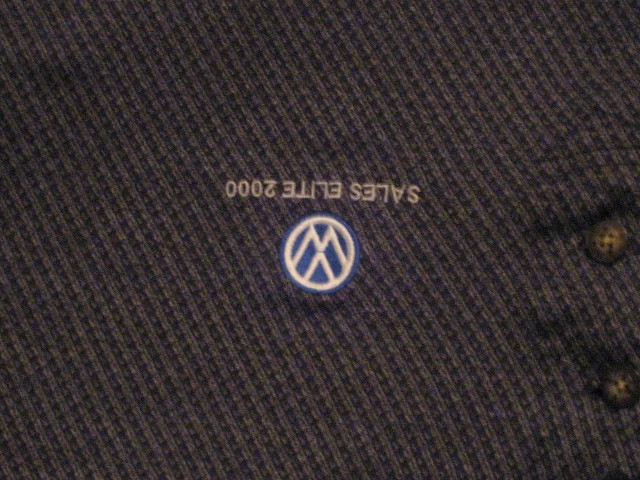This close-up photograph features an intricately embroidered Volkswagen emblem on a piece of fabric. The emblem, presented upside down, consists of the iconic circular "VW" logo with the text "Sales Elite 2000" stitched above it, also inverted. The embroidery is rendered in an off-white thread, providing a stark contrast to the dark gray fabric backdrop. The fabric itself is characterized by a crisscross hatch pattern with even darker stripes interwoven. On the right side of the image, there is a noticeable crease where the neckline would naturally form, accompanied by two brown buttons with four holes each, aligned vertically one above the other. Additionally, a longer, horizontal crease traverses the top of the photo, while another crease is visible on the left side, adding texture and depth to the fabric’s appearance.